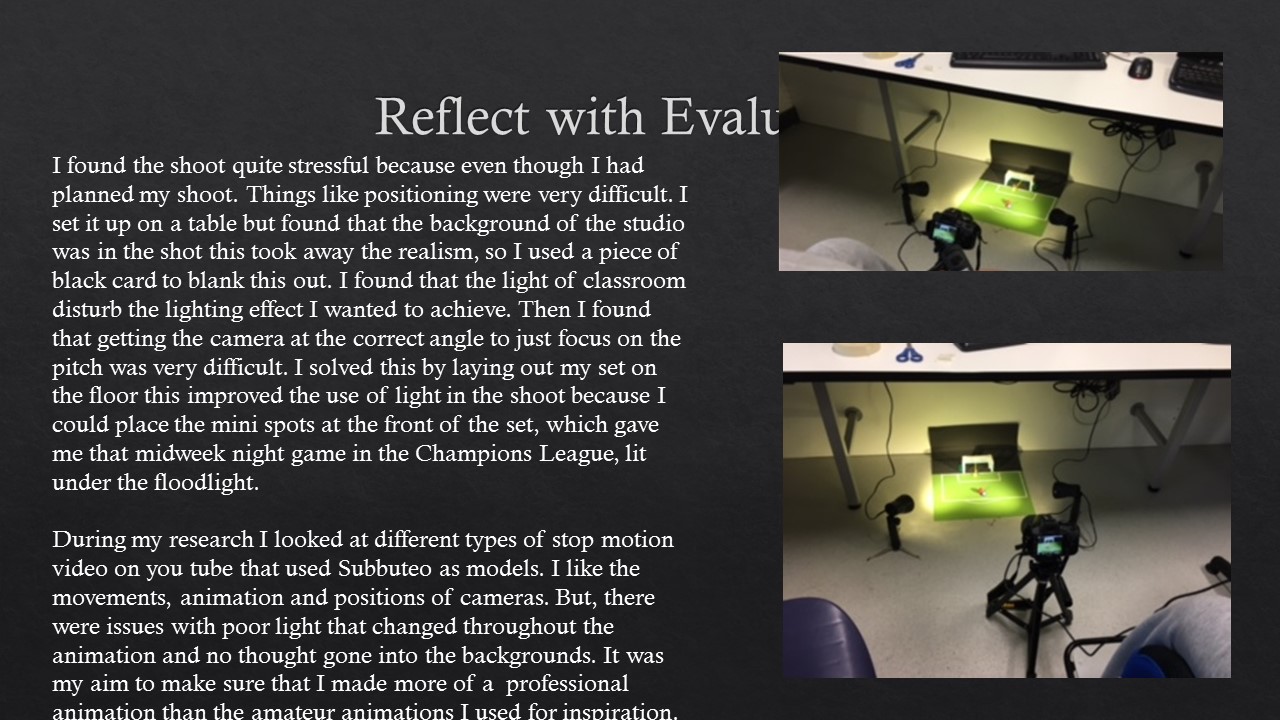The image is a detailed landscape-oriented photograph, wider than it is tall, featuring a miniature soccer field carefully arranged on a table. The scene is illuminated with specialized lighting, creating an effect reminiscent of a midweek night game in the Champions League under floodlights. At the back of the miniature field is a goal, and positioned in front of it is a red figurine, likely representing a player. Surrounding the miniature setup are various lights and a camera, which the photographer struggles to align perfectly to capture the desired angle and focus solely on the pitch.

In the background, a plain black card has been strategically placed to block out elements of the studio, enhancing the realism of the scene by removing distracting background details. The left side of the image is occupied by white text without indentation, which narrates the photographer's challenges and solutions throughout the shoot process. The text starts with the partially covered phrase "reflect with e-value" and comprises two paragraphs. The first paragraph details the photographer's stressful experience due to difficult positioning and lighting issues exacerbated by the setup being initially on a table. To rectify this, black card was used to mask the studio background, and eventually, the set was laid out on the floor to better manipulate the lighting.

The second paragraph highlights the photographer's research process, which involved studying various stop-motion videos on YouTube that utilized Subbuteo models. This research inspired a professional approach aimed at surpassing the amateur animations studied, focusing on consistent lighting and thoughtfully designed backgrounds.

Underneath the main image, a smaller inset photo shows the same miniature field from a different angle, reinforcing the detailed setup and lighting arrangement described in the photographer's narrative.